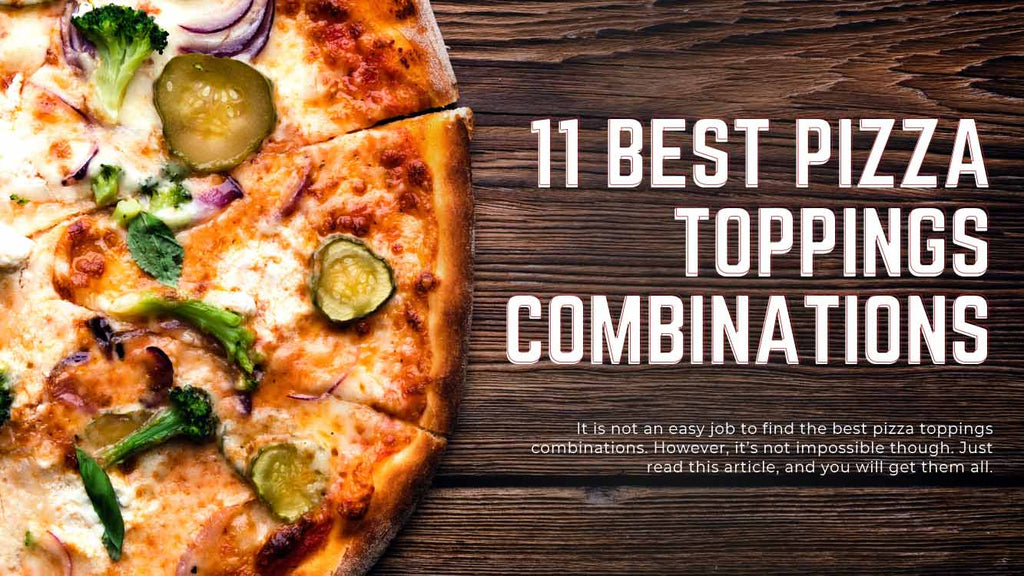This image features a partially visible pizza on the left side of the frame, displaying about three triangular slices that include toppings such as broccoli, sliced pickles, red onions, and melting cheese in various shades of yellow, cream, and golden brown. The crust of the pizza is a slightly darkened golden brown. The background of the image is a fake wood texture with visible grain, providing a rustic feel. On the right side of the picture, there is prominently displayed bold white text reading "11 Best Pizza Topping Combinations." Beneath this, in smaller white print, the text continues, "It is not an easy job to find the best pizza toppings combinations. However, it's not impossible though. Just read this article and you will get them all." This detailed description suggests that the image itself serves as an advertisement or promotional material touting unique pizza topping combinations.